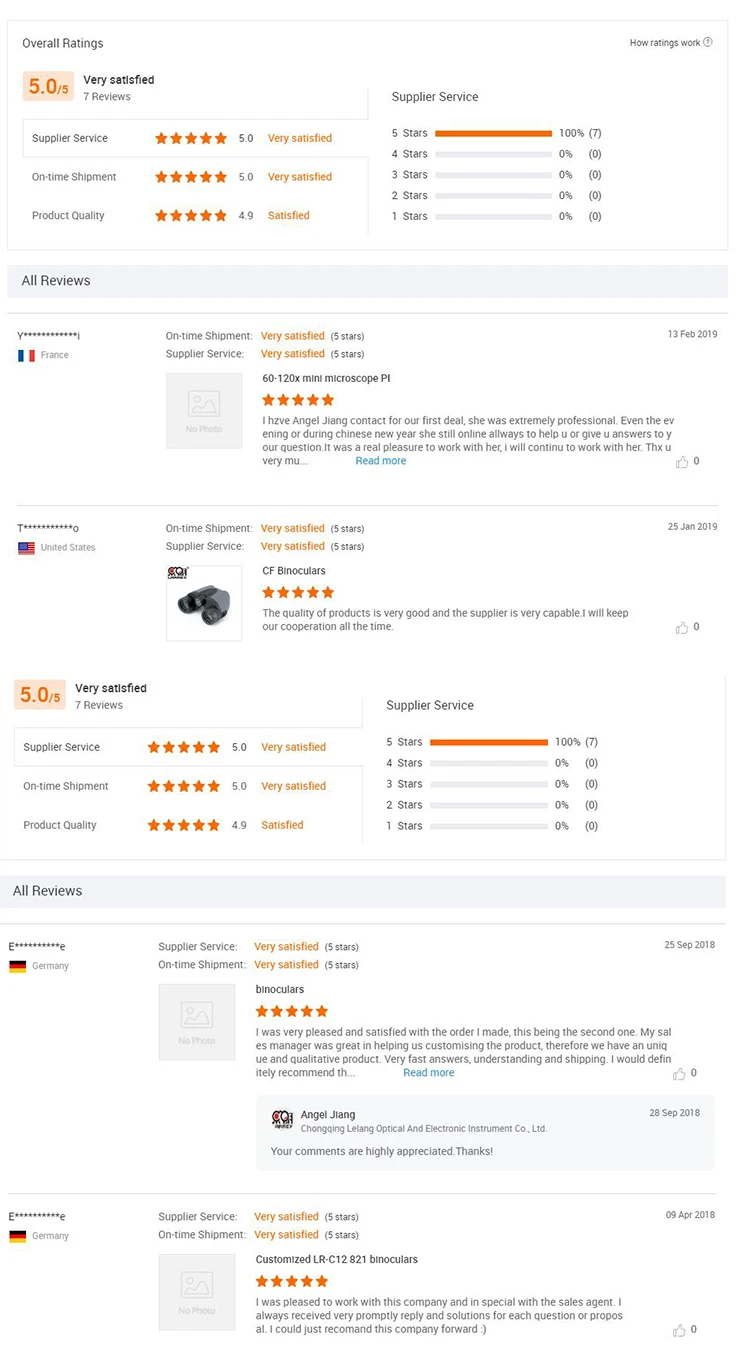The image is a screenshot displaying ratings and reviews for multiple products. The primary title at the top left corner of the image reads "Overall Ratings." The first rating beneath this title indicates that the service received a "Very Satisfied" rating of 5.0 out of 5. It appears to be related to supportive service, likely an online service, although the text is somewhat merged and difficult to read clearly. Another section shows that the product quality received a rating of approximately 4.9, labeled as "Satisfying." Below these summary ratings, there are more detailed written reviews and additional ratings.